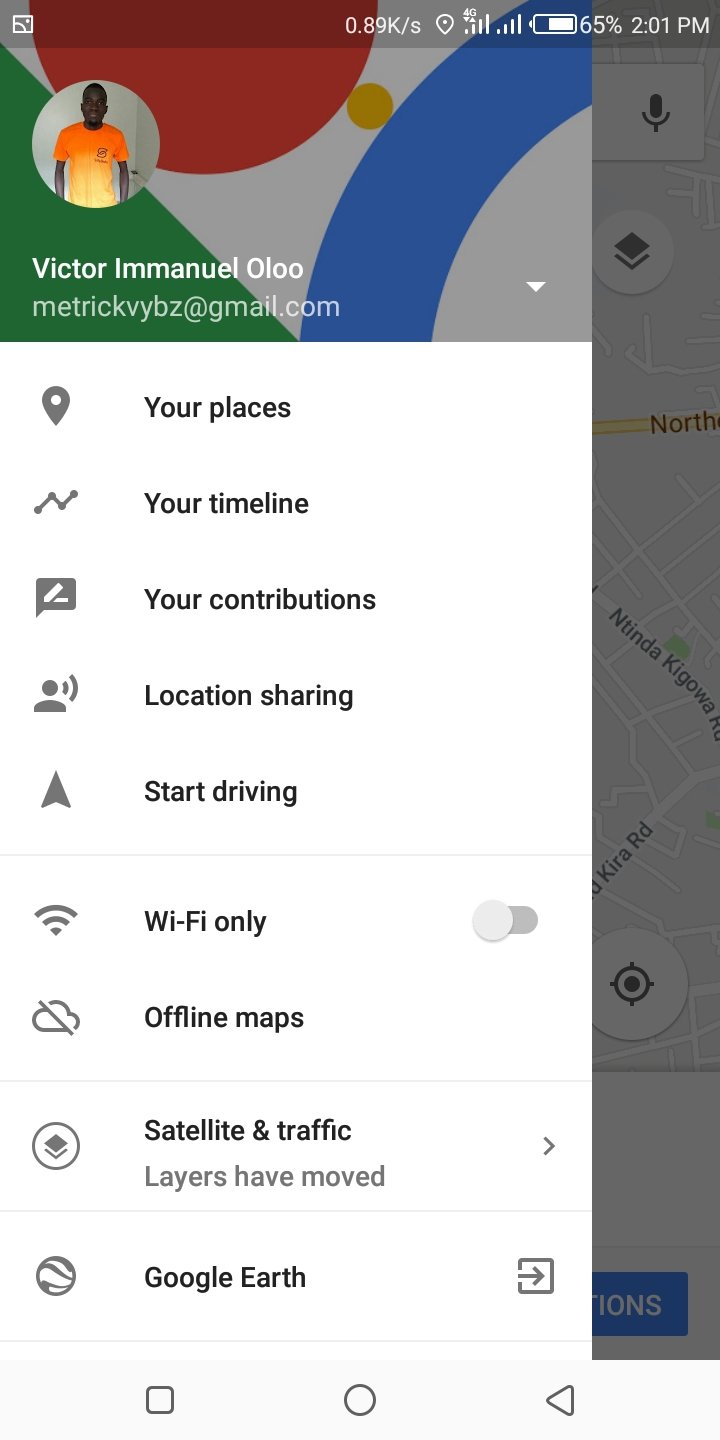The image showcases a series of screenshots captured from a mobile device. In the top right corner, there are several indicators: the network speed meter, a location icon, and icons for SIM 1 and SIM 2, with SIM 1 currently active and connected to 4G. The battery level is at 65%, and the device displays the time as 2:01 PM.

The device is logged in with the name "Victor Emmanuel Oluo," using the email "metricbybz.gmail.com." The interface visible in the screenshots includes various options such as "Your places," "Your timeline," "Your contributions," "Location sharing," and "Start driving." Additional options mentioned are "Wi-Fi only," "Offline maps," "Satellite and traffic," and "Layers have moved." A Google Earth exit option is also noted.

Navigation buttons are located at the bottom of the screen: the "Recent apps" button is on the left, the "Home" button is in the center, and the "Back" navigation key is on the right. In the background, a map interface is visible, which appears to be disabled.